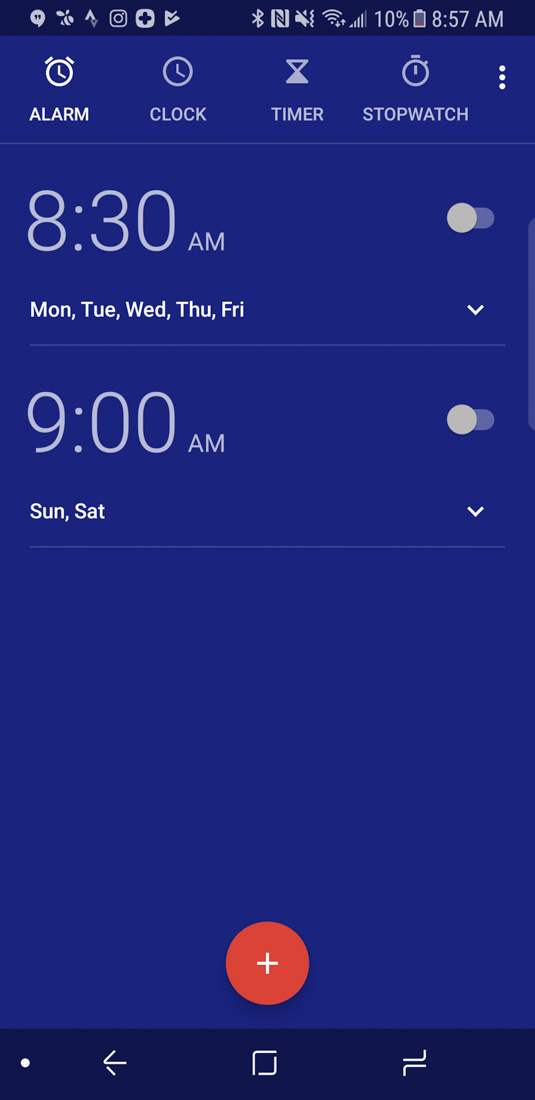The image depicts a smartphone screen displaying an alarm management interface. At the top, a black status bar indicates the time as 8:57 AM and shows the battery life at a critical 10%, along with various other indeterminate icons. Below this, the screen has a midnight blue background. Along the top, from left to right, are icons for different time-related functions: an alarm clock, a regular clock, a timer, and a stopwatch.

Two alarm times are listed beneath these icons. The first alarm is set for 8:30 AM, labeled for Monday through Friday, but it is toggled off. The second alarm is set for 9:00 AM, designated for Saturday and Sunday, and it is also toggled off. At the very bottom of the screen, there is an orange circular button with a white plus sign in its center, likely for adding a new alarm. Directly below this is a navy blue navigation bar featuring a back button, a home button, and a refresh button.